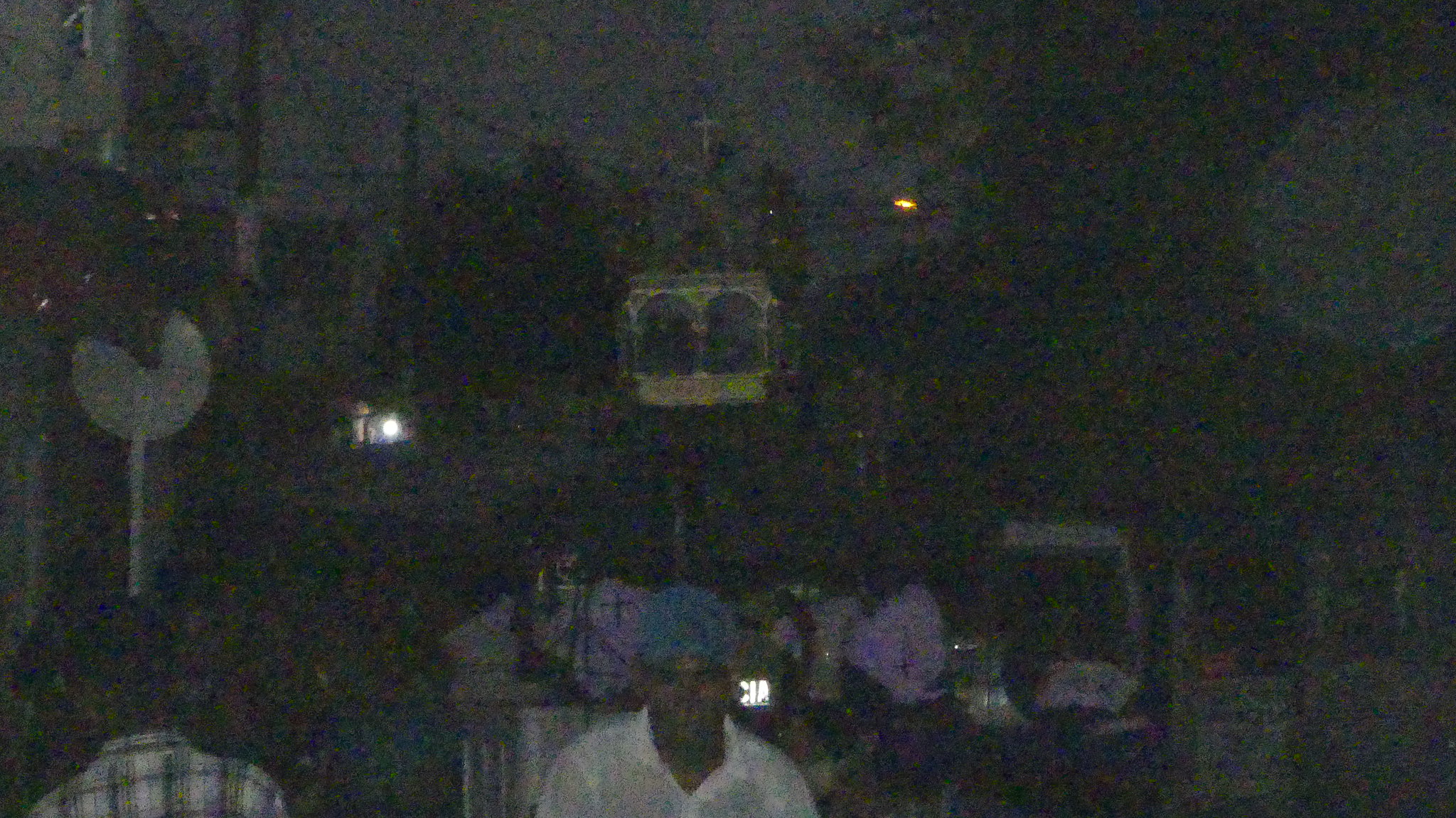This grainy photograph captures a nighttime scene at what appears to be a gathering, possibly a party or a church event, given the visible white cross in the background. The overall image quality is very poor, with significant splotchiness and darkness making details hard to discern. The setting seems to be a neighborhood with some visible trees, particularly a large cluster on the right side of the image in the upper portion.

In the foreground, slightly towards the center, stands a black gentleman wearing a blue hat and a white shirt. Behind him are several individuals draped in robes adorned with crosses, suggesting a religious affiliation. To the left of the central figure, another thin black man is seen facing away from the camera, wearing a plaid shirt. The photograph's poor quality evokes a sense of mystery, likened to historic, distressed images.